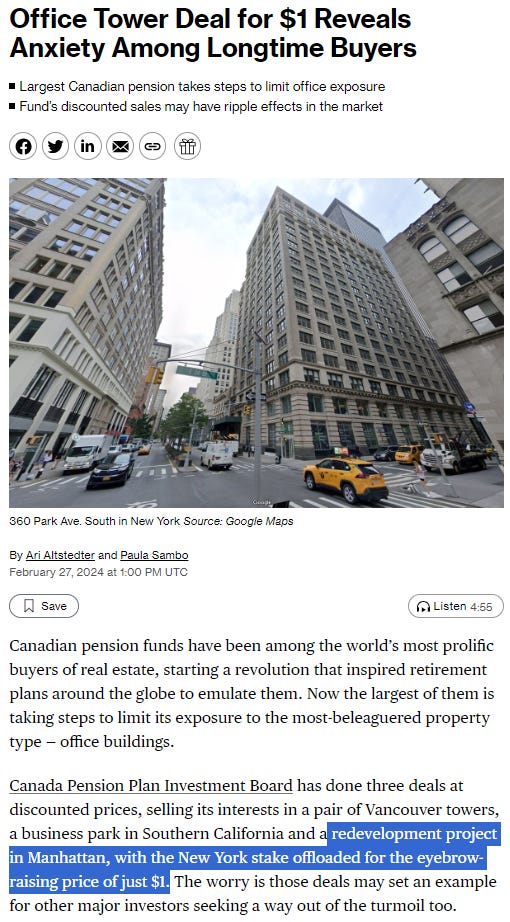**Office Tower Deal for $1 Reveals Anxiety Among Longtime Buyers**

---

Largest Canadian pension takes steps to limit office exposure  
Funds' discounted sale may have ripple effects in the market

---

![Image of a cityscape](https://www.google.com/maps/@3060ParkAvenueSouthNewYork)

**Source:** Google Maps

*By Arie Austaditter and Paula Sembo, [Date]*

---

**Save** | ![Headphones icon] Listen

---

Canadian pension funds have been among the world's most prolific buyers of real estate. Recently, a redevelopment project in Manhattan, located at 3060 Park Avenue South in New York, was offloaded for the eyebrow-raising price of just $1. This decision raises concerns about the future market stability.

---